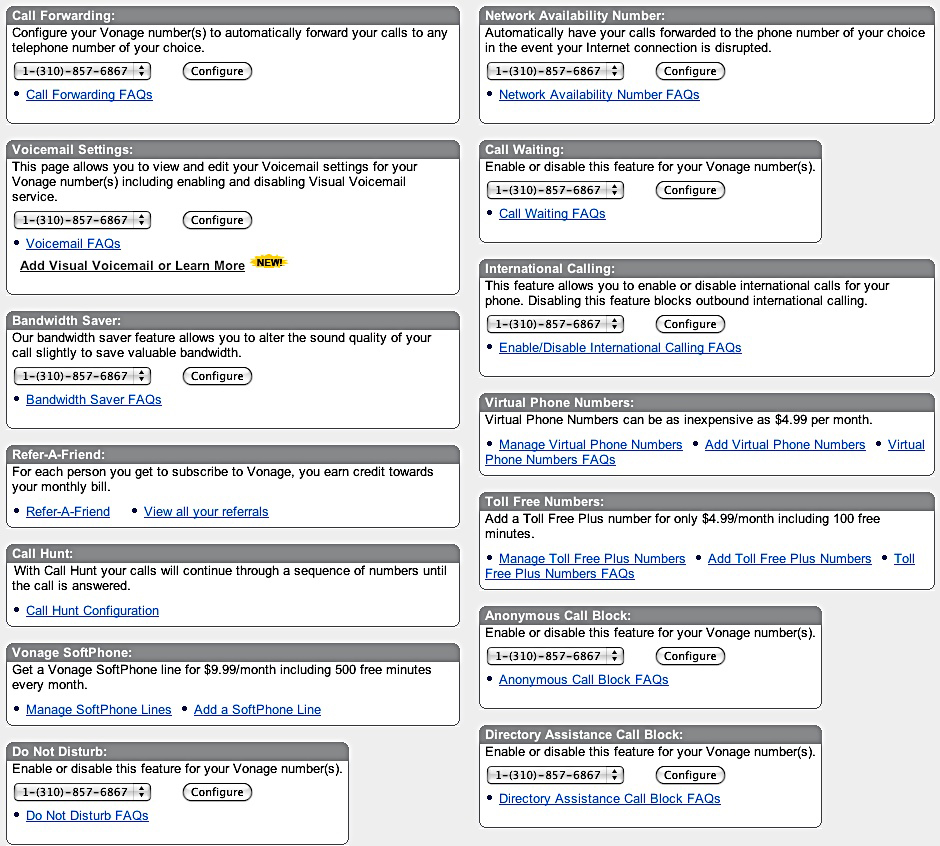The image showcases a detailed guide for configuring various features of a Vonage phone service. The guide is organized into two columns of seven rectangular boxes each, making a total of fourteen boxes. Each box contains a gray header with a feature title written in black text, followed by descriptions and hyperlinks in blue.

On the left side, the boxes describe the following features:

1. **Call Folder** - Automatically directs your calls to the telephone number of your choice.
2. **Voicemail Settings** - Allows you to view and edit your voicemail settings, including enabling the Visual Voicemail service for your Vonage number.
3. **Bandwidth Saver** - Adjusts the sound quality of your calls to conserve bandwidth.
4. **Refer a Friend** - Encourages you to invite others to subscribe to Vonage, earning credit towards your bill.
5. **Call Hunt** - Your calls progress through a sequence of numbers until answered.
6. **Vonage Cell Phone** - Offers a cell phone line at $9.99 per month, including 500 free minutes.
7. **Do Not Disturb** - Allows you to enable or disable this feature for your Vonage number.

On the right side, the boxes cover these features:

1. **Network Availability Number** - Automatically forwards calls to another number if your internet connection is disrupted.
2. **Call Waiting** - Enables or disables the call waiting feature for your Vonage number.
3. **International Calling** - Controls the ability to make international calls, with an option to block outbound international calls.
4. **Virtual Phone Numbers** - Available for as little as $4.99 per month.
5. **Toll-Free Numbers** - Add a toll-free number for $4.99 per month, which includes 100 free minutes.
6. **Anonymous Call Block** - Enables or disables the ability to block anonymous calls for your Vonage number.
7. **Direct Assistance Call Block** - Enables or disables the feature to block direct assistance calls for your Vonage number.

The consistent template of each box, featuring the number "1" and area code "310-857-6867," reinforces the instructions' uniformity and clarity. The blue hyperlinks adjacent to "Configure" in most boxes provide further customization options for each feature.